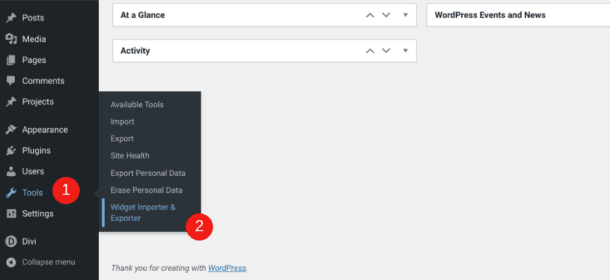The image depicts a webpage with a predominantly dark theme. On the left-hand side, there is a vertical navigation bar with a black background listing various menu items such as "Posts," "Media," "Pages," "Comments," "Projects," "Appearance," "Plugins," "Users," "Tools," "Settings," and an item partially labeled "Collegiate something" at the bottom. Next to "Tools," which is marked by an icon resembling tools, there is a red circle with the number "1" inside it, indicating a notification.

The main content area of the webpage has a light gray background. Within this area, there is a white box labeled "At a Glance," featuring up and down arrow icons that suggest collapsible or expandable content. Similarly, another white box labeled "Activity" also includes up and down arrows. In the top right corner of the main content area, the webpage displays "WordPress Events and News" in black lettering.

Outside the dark vertical navigation bar, there is a black pop-out sidebar containing additional options such as "Import," "Export," and "Site Health." The highlighted option within this sidebar is the bottom one, which has a red circle with the number "2" inside it, indicating another set of notifications.